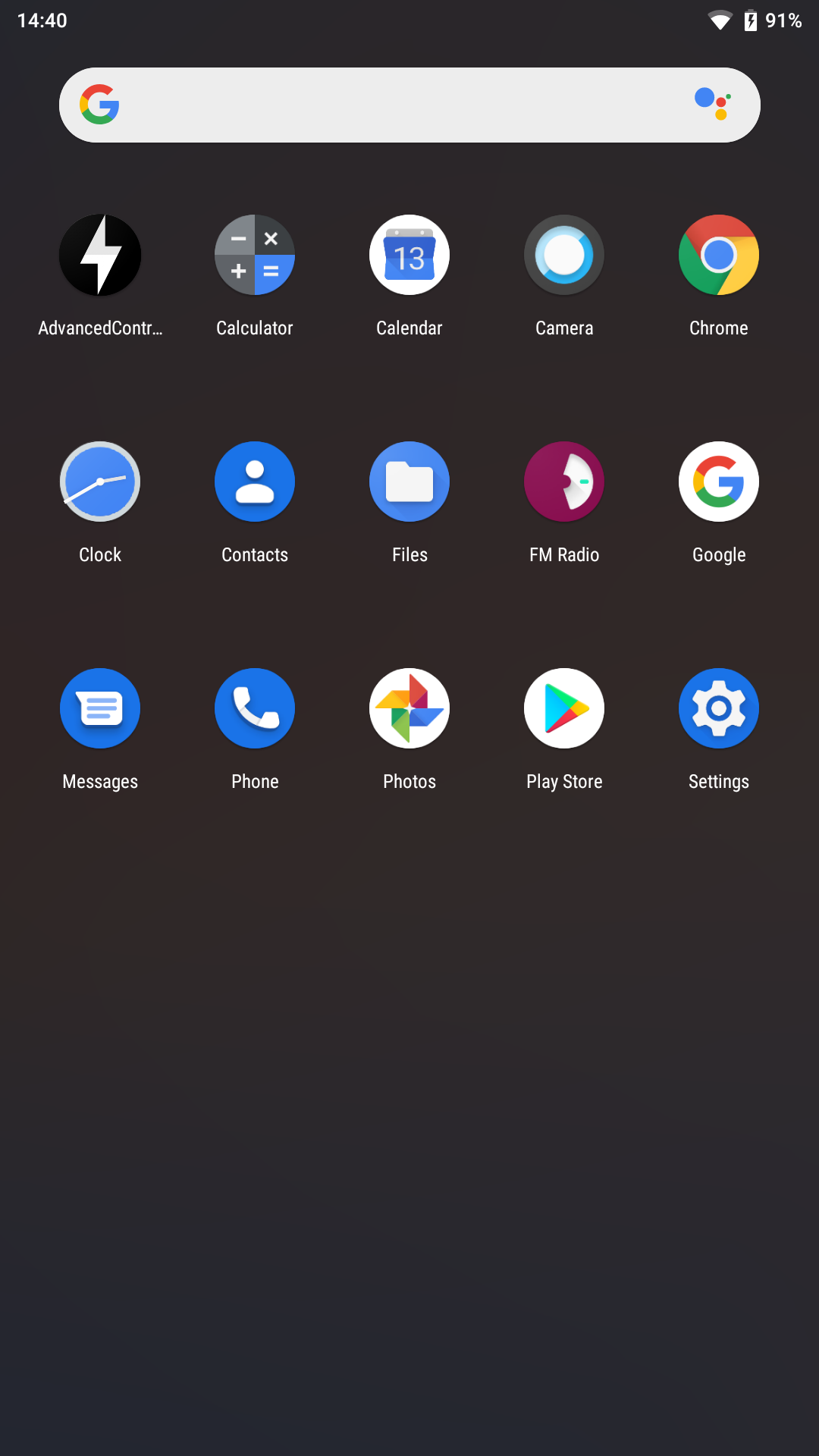This is a detailed screenshot of the app drawer on an Android smartphone, possibly a OnePlus or Google Pixel device. The background is a dark, opaque gray, providing a sleek contrast to the vibrant app icons. In the top left corner, the current time is displayed, and in the upper right corner, there are indicators for signal strength and battery life.

Just below these indicators is a Google search bar, with the recognizable "G" logo in red, yellow, green, and blue on the left side. Adjacent to the logo, a series of colorful dots—blue, red, yellow, and green—likely represents the voice assistant activation icon.

The app drawer itself consists of three rows with five app icons each, neatly organized and labeled. The apps visible include: Advanced Control, Calculator, Calendar, Camera, Chrome, Clock, Contacts, Files, FM Radio, Google, Messages, Phone, Photos, Play Store, and Settings. Each app icon is accompanied by a small circular symbol corresponding to its respective application.

Given the basic range of pre-installed apps, it appears that this is either a brand new device or one that has been recently reset to factory settings. The overall color palette is subdued, highlighting the colorful app icons against the dark background for improved visibility and aesthetic appeal.